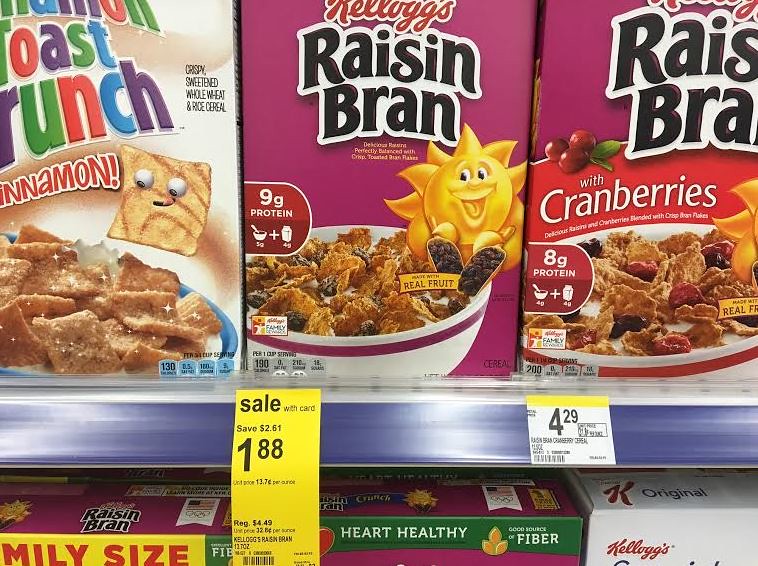In this detailed close-up photograph taken in the cereal aisle of a grocery store, the image prominently features a variety of cereal boxes stacked on two visible shelves. On the top-left corner, a box of Cinnamon Toast Crunch is displayed, complete with a glimpse of its playful cinnamon toast cereal mascot. Beside it, at the center, sits a box of Kellogg's Raisin Bran, showcasing 9 grams of protein and accompanied by an eye-catching yellow sale tag that reads, "Sale with card: Save $2.81, $1.88, regular $4.49." To its right, there's a box of Kellogg's Raisin Bran with Cranberries, marked at $4.29, boasting 8 grams of protein and an assertion that it's made with real fruit. Just below, on the lower shelf, one can partially see additional cereal boxes, including Raisin Bran, Raisin Bran Crunch, and Kellogg’s Original. The lower shelf reveals varied hues of purple, red, green, blue, white, and brown, hinting at the diverse selection of cereals barely visible in the image's bottom edge. The scene is rich with vibrant packaging, nutritional labels, and multiple pricing details, capturing the essence of a bustling grocery store cereal aisle.